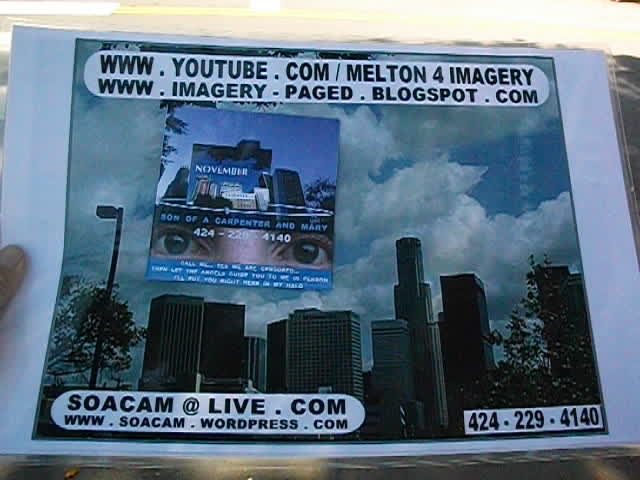The image depicts a printed advertisement being held, with a visible thumb on the left side. The central image features a cityscape consisting of tall skyscrapers, surrounding trees, and a street light against a backdrop of a blue sky filled with white clouds. Superimposed on this scene is an inset of a closely zoomed-in pair of dark brown eyes, with the text “November” printed above them and a phone number, 424-229-4140, overlaid in white.

At the top of the printout, there's a YouTube link, "www.youtube.com/MeltonForImagery," and a blog link, "www.imagery.page.blogspot.com." Additional links at the bottom include "soacam@live.com" and "www.soacam.wordpress.com." The text appears in a standard black font against white backgrounds, making the URLs and contact information stand out clearly. The arrangement suggests that the advertisement is intended to draw attention to various online resources, but its purpose remains unclear, possibly implying it is a scam.